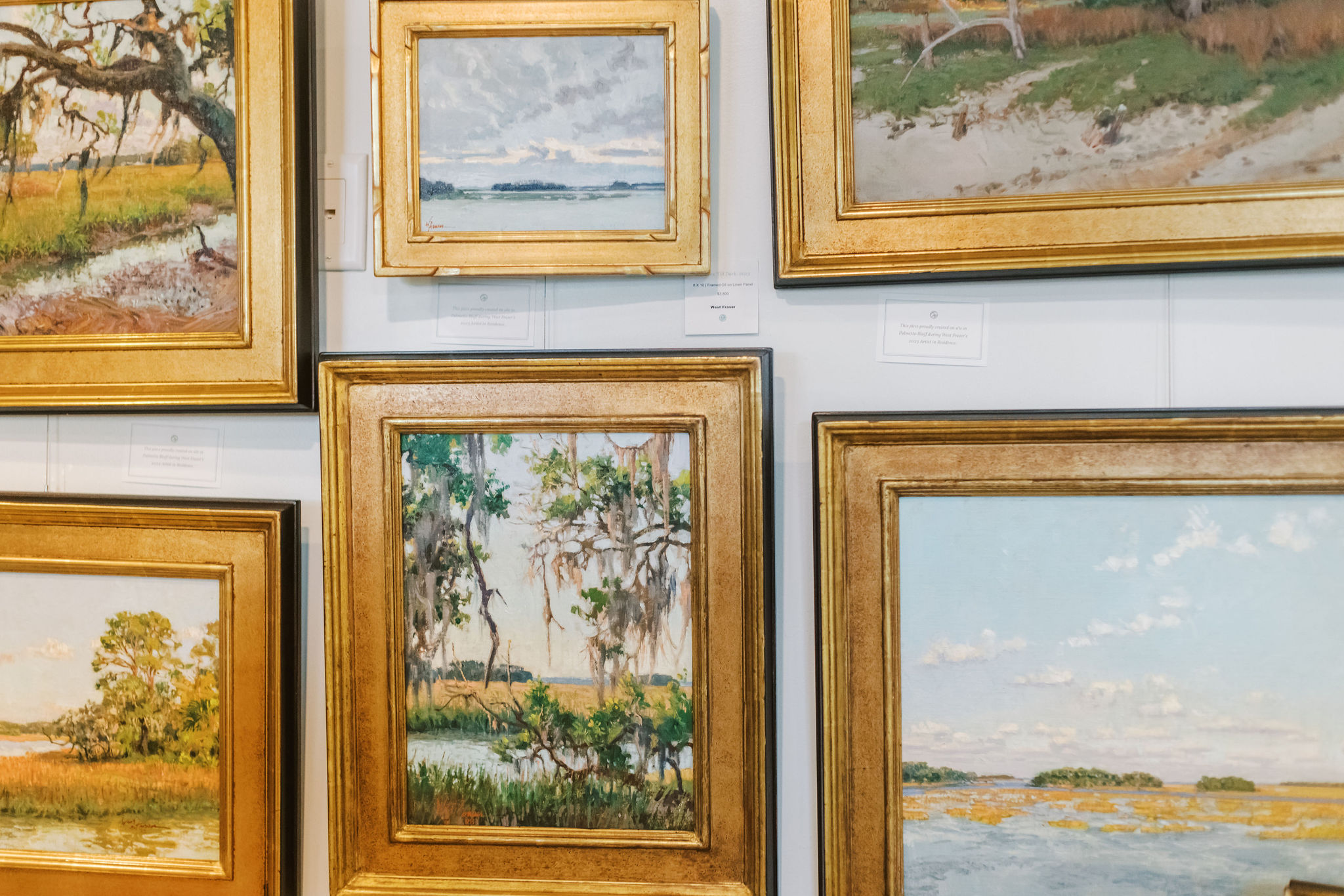A photograph showcases six paintings displayed on a museum wall, each in a golden frame. These landscape paintings predominantly feature scenes of nature, particularly marshlands or possibly the Everglades in Florida. The central painting, fully visible, depicts Spanish moss hanging from tree limbs over a waterway, likely a river or large creek, with a field in the background. Similarly, the painting in the upper left corner, cut off at the edges, echoes this theme with Spanish moss, golden grasses, and a body of water. The upper middle painting displays a tranquil sky, while the lower right painting reveals a river with plants. All six paintings, positioned around a central piece and accompanied by descriptive cards, are mostly landscapes showcasing serene natural settings, although some are partially obscured by the photograph's frame.